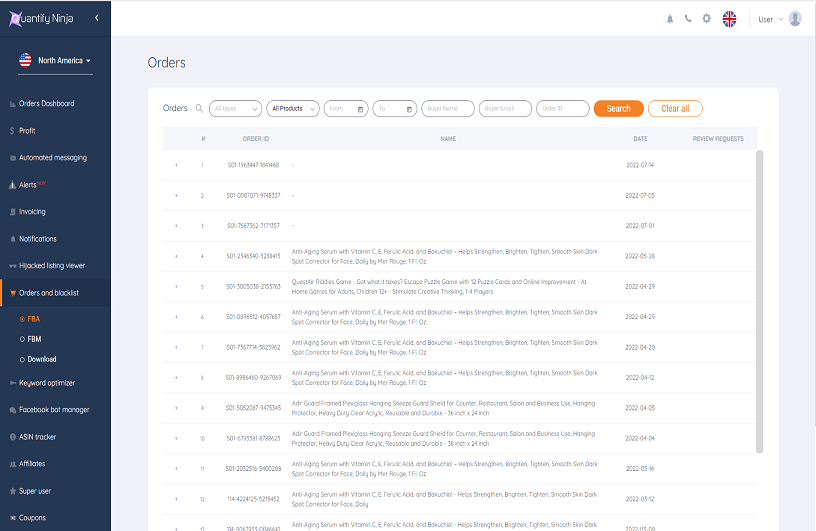This is a comprehensive screenshot of the Quantify Ninja website interface. In the upper left corner, "Quantify Ninja" is prominently displayed. Along the left-hand side of the screen, there is a vertical navigation menu. The first entry reads "North America," accompanied by a drop-down menu icon and a small American flag within a circle. Below this, red-lettered entries include "Orders," "Dashboard," "Profit," "Automated Messaging," and "Alerts." Other notable sections include "Hijacking Notifications," "Hijacked Listing Viewer," "Order and Block List," "FBA," "FBM," "Download Keyword Optimizer," "Facebook," "Bot Manager," "ASN Tracker," "Affiliates," "Super User," and "Coupons." 

On the right side of the screen, the main content area displays an "Orders" screen. The top of this section features a navigation bar with "Orders" and several filtering options labeled "All Types," "All Products," "From," and "To," followed by "Fire Home" and "Fire Email." Beneath these options, the order list begins with product entries such as "Anti-Aging Serum with Vitamin C, E, Folic Acid." The detailed interface elements and functionalities provide a thorough overview of the Quantify Ninja website screenshot's features.